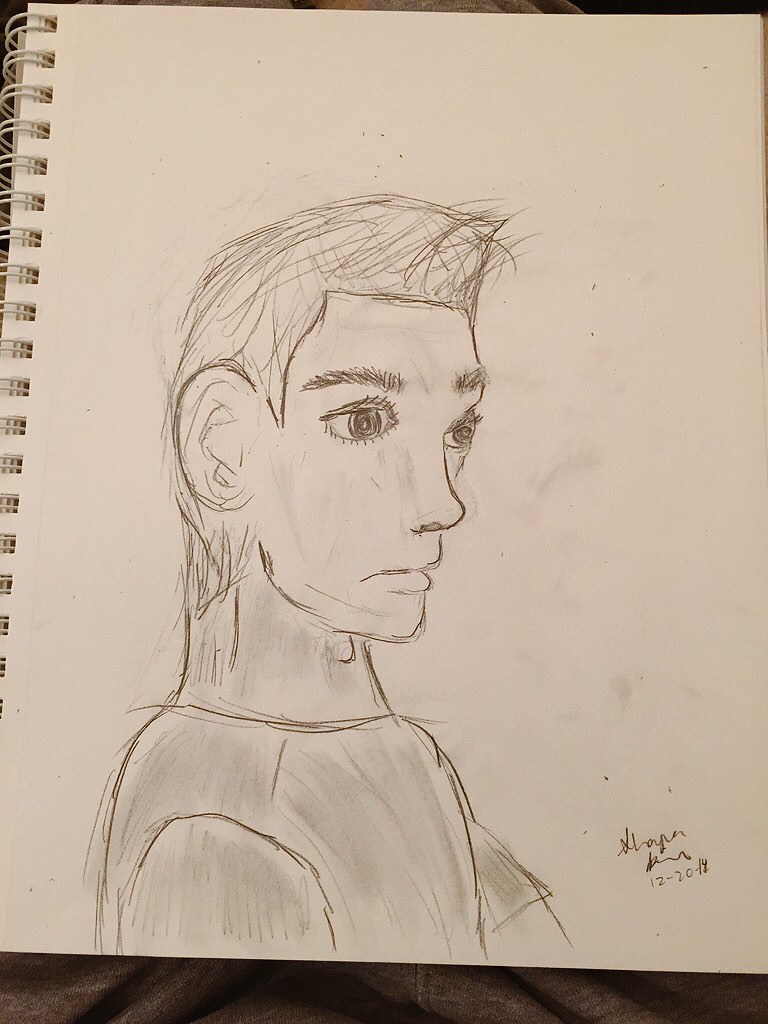In the photograph, there's a wrinkled purple fabric, possibly a bed sheet, serving as the background. Placed on this fabric is an open spiral-bound sketchpad displaying a detailed pencil sketch. The drawing, done on a light gray paper, portrays a young man in profile, facing to the right, with a neutral expression. The man's features include short hair, bushy eyebrows, large eyes, and prominent ears. He is depicted from the shoulders up, wearing a short-sleeved shirt. The artist's signature and the date "12-20-2014" are inscribed on the bottom right corner of the page, the signature being illegible.